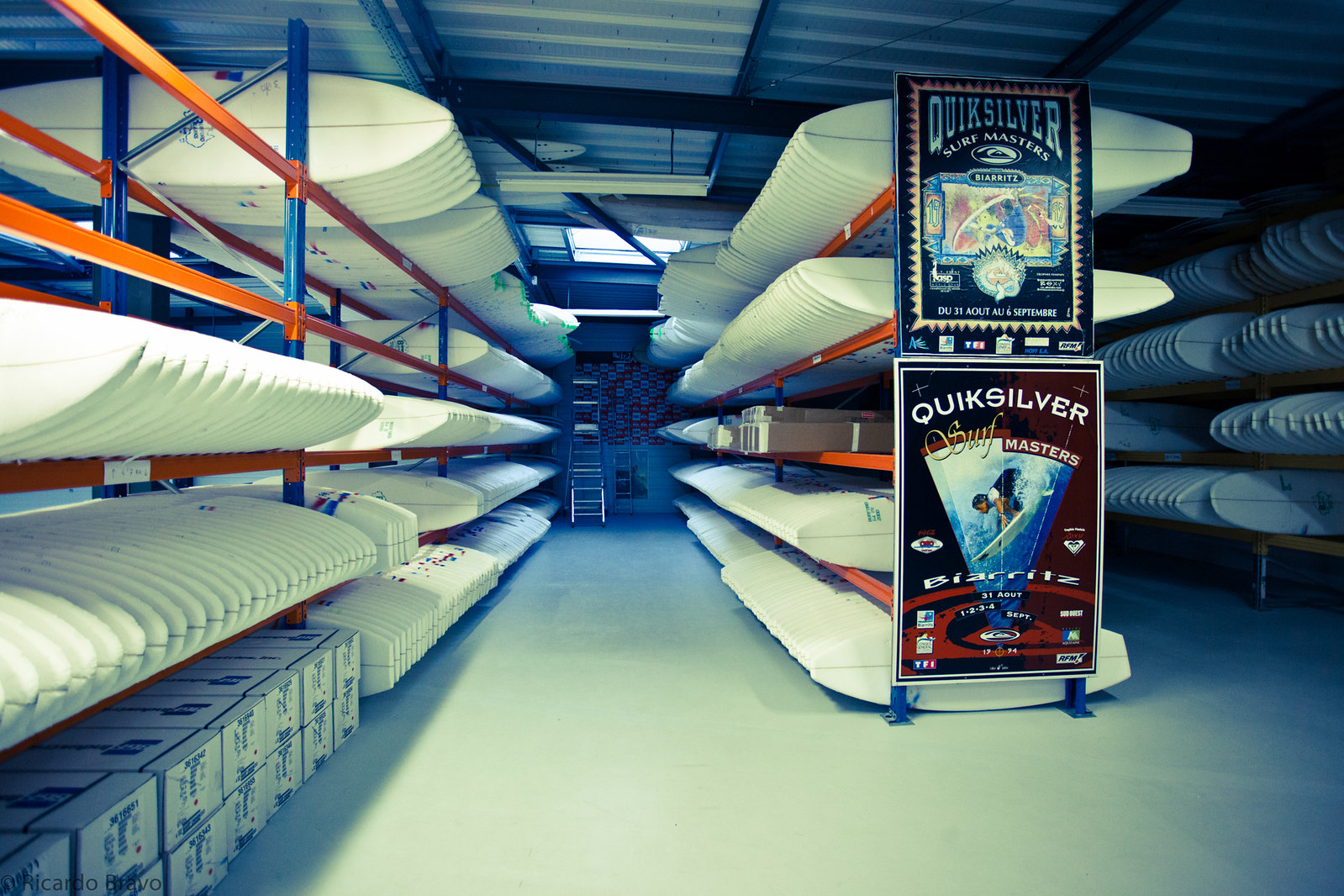This photograph captures the interior of a warehouse, illuminated by natural light streaming through a moonroof while fluorescent lights remain off. Central to the image are metal shelves with blue posts and horizontal orange rails, neatly stacked with white surfboards placed sideways. Two prominent posters are affixed to the end of one shelf: the top one is a blue "Quicksilver" poster, while the bottom is a red "Quicksilver Surf Masters" poster, featuring an image of a surfer about to ride a wave. At the far end of the warehouse, a six-foot ladder stands against a wall. The white-tiled floor adds to the warehouse's clean and organized appearance.